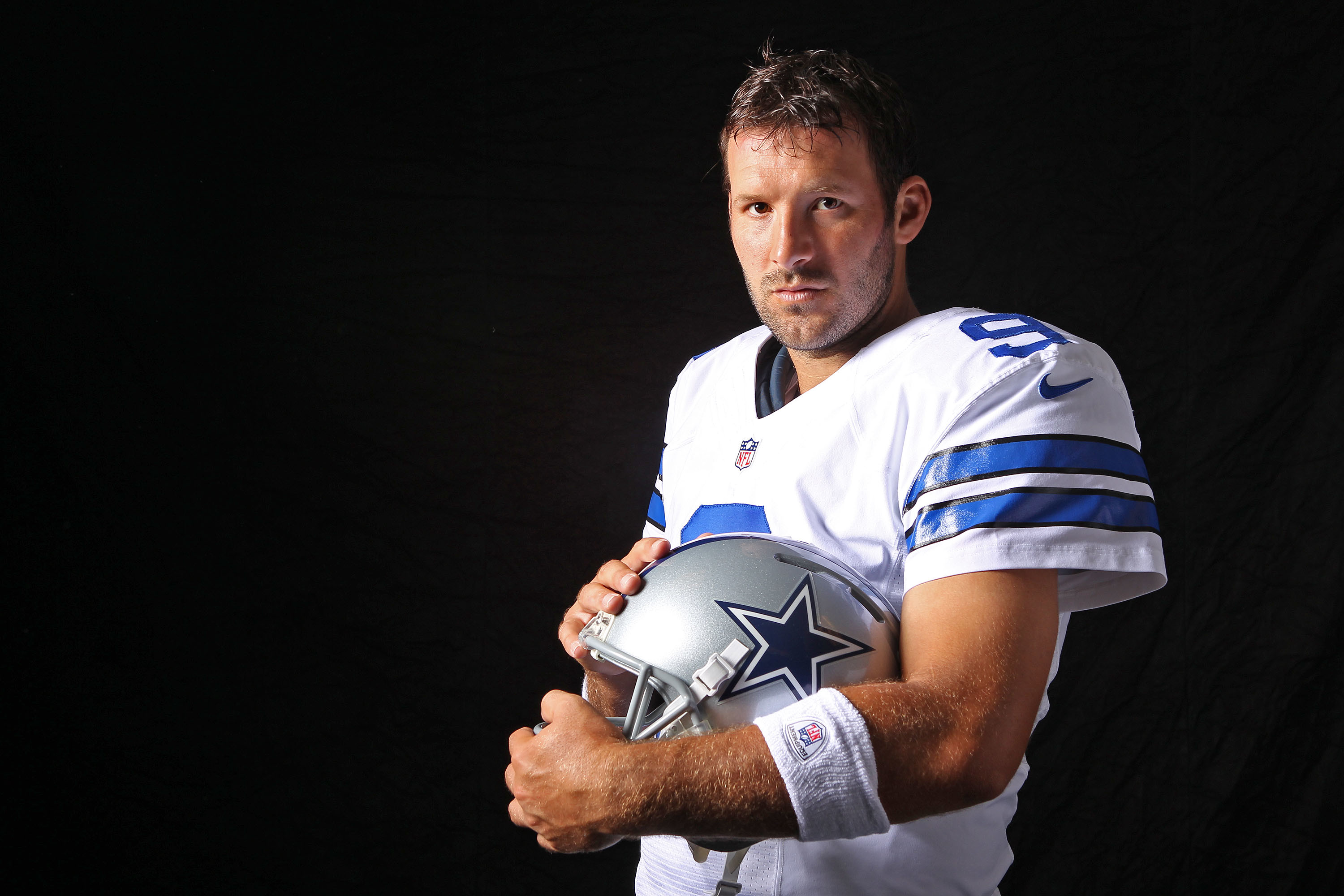The photograph captures Tony Romo, the retired quarterback of the Dallas Cowboys, in a dramatic, black-void setting, emphasizing his serious, all-business demeanor. He is presented from the waist up, with his body angled towards the bottom left corner, while his face stares intensely straight into the camera, marked by a rugged five o'clock shadow and tousled hair, suggesting a practice session. Romo is dressed in the iconic white Dallas Cowboys jersey, featuring blue stripes on the sleeves and the prominent number nine on the chest and shoulders. Beneath his jersey, the black and blue padded protection is visible, indicative of his readiness for the game. He holds a silver helmet with a grey face guard, emblazoned with the Cowboys star, close to his chest with both hands. A white sweatband with a SHIELD logo encircles his forearm, adding a touch of functionality and detail to his gear. The entirely black background gives the impression of a studio photo shoot, focusing all attention on Romo's imposing presence.